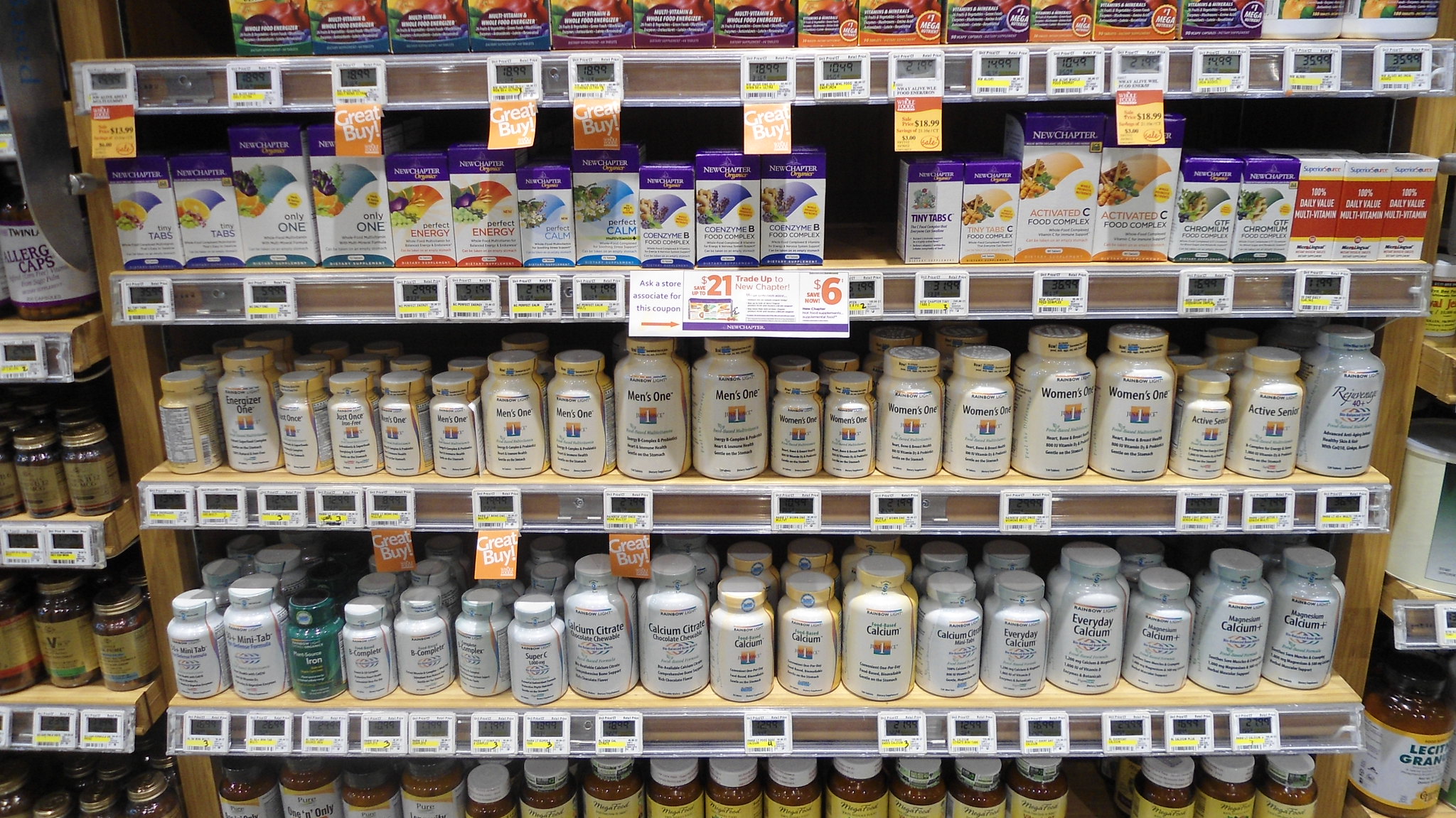A meticulously organized wall of vitamins and supplements in a health food store is showcased on a series of shelves crafted from light-colored wood. The display consists of five tall shelves, beginning from the lower shelf up to the top. Each shelf is lined with digital price signs encased in white plastic housing. Prominent among the tags are a few red labels with white lettering that read "Great Buy," indicating special offers on certain multivitamins.

The assortment includes a variety of products such as women's and men's one-a-day vitamins, calcium supplements, and other health aids, all packaged in white bottles featuring a square logo. Although the logo is slightly blurry, it appears to depict a white pillar or the number one. These bottles are characterized by their cream-colored neckbands securing the lids. Some bottles are purely white, while others sport a combination of white and yellow.

Additionally, the top two shelves are home to a row of square supplement boxes. With its neatly arranged and clearly labeled products, the scene unmistakably suggests a health food or grocery store dedicated to wellness and nutrition.